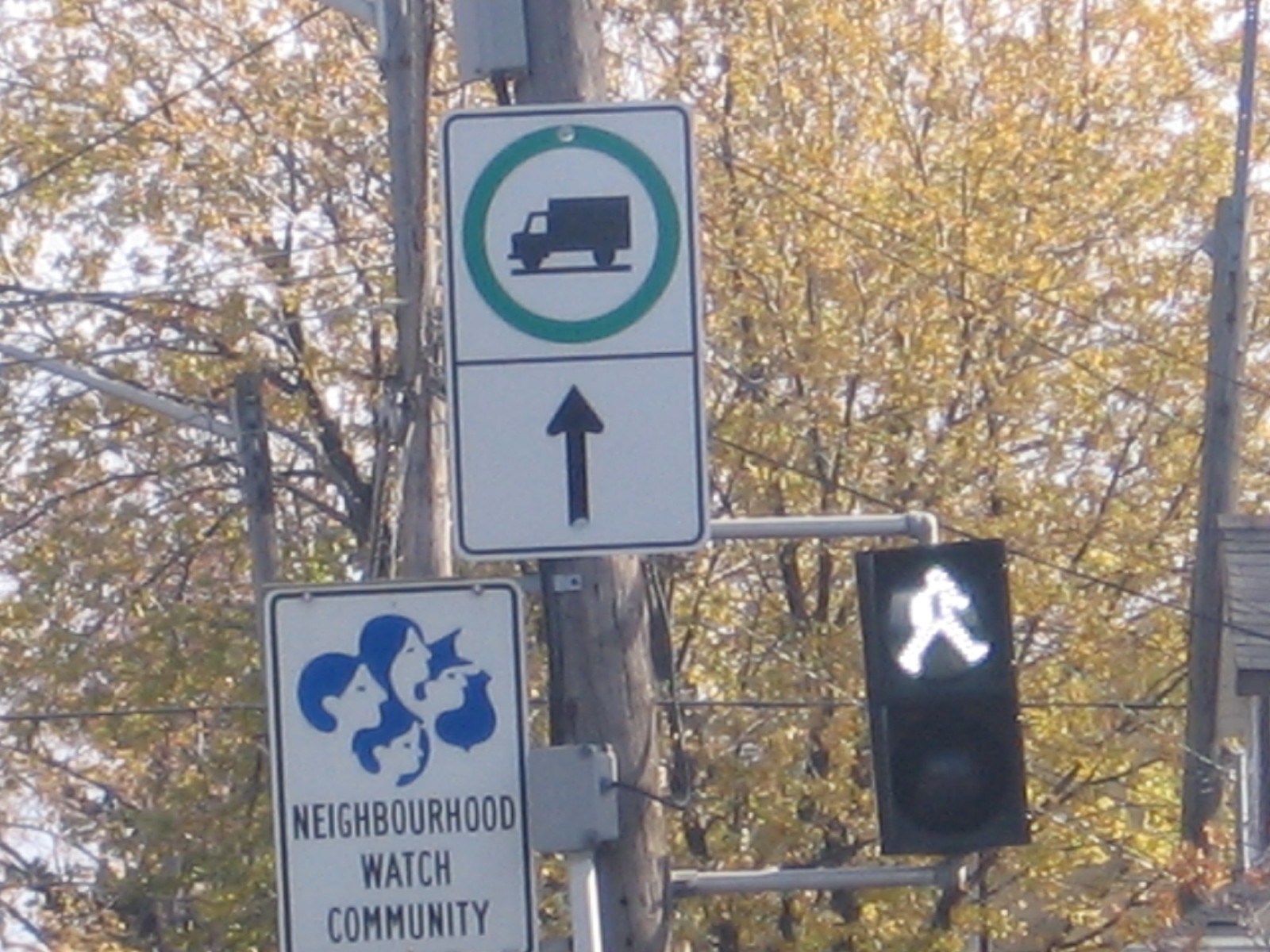The photograph is a vivid, full-color outdoor scene, captured during daytime in what appears to be fall, signaled by the vibrant yellows and oranges of the leaves on the several trees in the background. A patchy, gray sky peeks through the foliage, contributing to the autumnal atmosphere. On the far right side of the image, part of a home's roof and several phone lines are visible.

In the foreground, dominating the scene are street signs affixed to a pole. Prominently, there is a traffic signal displaying a bright white icon of a person walking, indicating a crosswalk. Above this signal is a rectangular white sign featuring a large green circle with a silhouette of a black truck inside it, and a black arrow pointing upwards towards the truck and circle. Just below this, another rectangular sign displays a blue illustration of four people accompanied by a police shield, with black text proclaiming "Neighborhood Watch Community." The overall composition vividly captures an intersection framed by community watch warnings and traffic guidance, set against the backdrop of a typical suburban neighborhood.